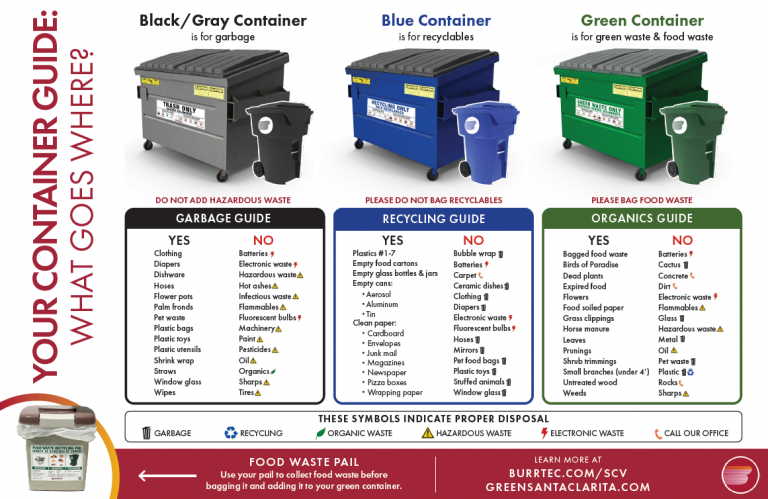The image is a detailed infographic serving as a comprehensive guide to trash, recycling, and organic waste containers. At the top, there are three prominently displayed containers aligned horizontally: a black/gray container for garbage, a blue container for recyclables, and a green container for organic waste and food scraps. Each container has a specific function clearly labeled. 

The black/gray container is designated for general garbage, suitable for items like clothing, diapers, dishware, and hoses, but explicitly forbids hazardous waste, electronics, and batteries. The blue container handles recyclables, including aerosol cans, aluminum, tin, cardboard, and envelopes, while excluding bubble wrap, batteries, carpets, and ceramics. The green container is for organic material such as bagged food waste and dead plants, prohibiting items like batteries, glass, and flammable materials.

On the left side of the infographic, in prominent red letters, the text "Your Container Guide: What Goes Where" emphasizes its instructional purpose. Below this text, the infographic elaborates with detailed "yes" and "no" lists for each type of container, providing examples of acceptable and unacceptable items. Additionally, there is a visual display of what a food waste pail looks like and a website link for more information. The colors used in the infographic include black, blue, green, red, orange, and gray, making it visually distinct and easy to follow.